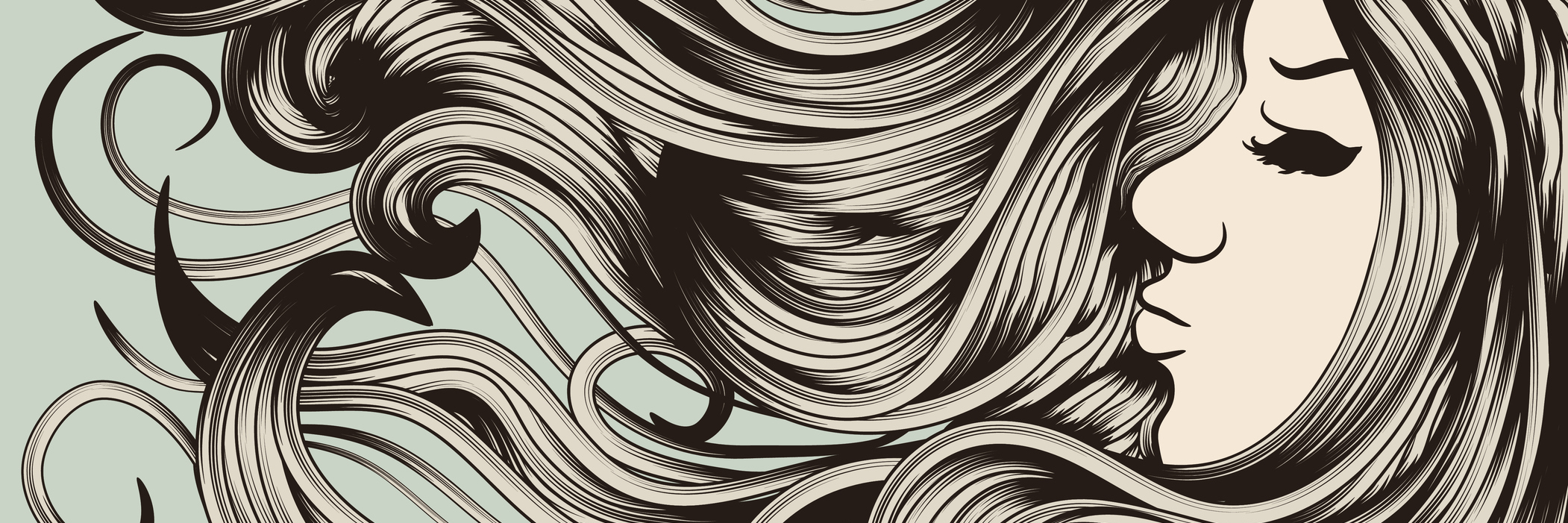This is a detailed black and white 2D illustration of a woman's face positioned in the right-hand corner of a long, landscape-oriented image with dimensions around 3 or 4 by 1. Her face is shown in profile, displaying a closed eye adorned with dark mascara and eye shadow, and a prominently curved black eyebrow. Her nose is rounded, and her full lips are shut. Her very long, flowing hair, depicted in black and grayish hues, extends horizontally from her head on the right all the way to the left edge of the image, with the tresses appearing wavy and almost wild as though moved by a strong wind. The background color is a subtle light blue, adding minimal color contrast to the predominantly monochromatic scheme of the illustration.